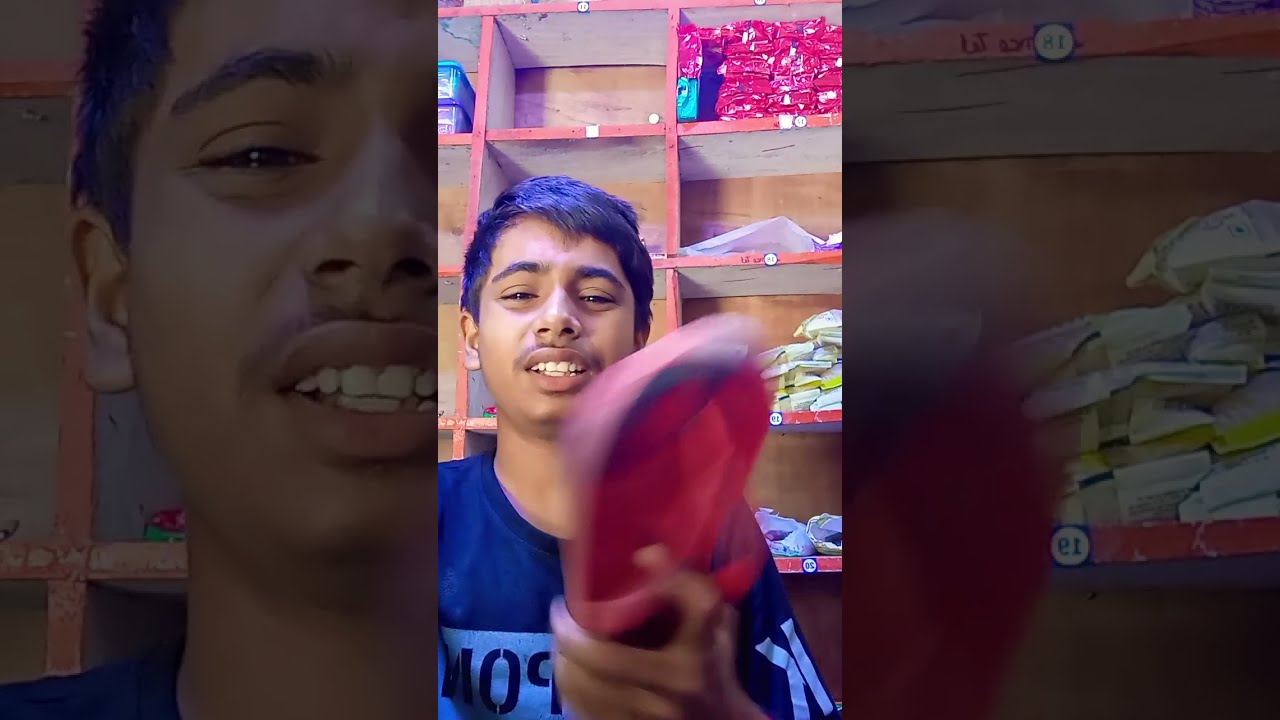In this image, we see a young man, likely around 15 or 16 years old, with a medium complexion and short black hair. He is wearing a navy blue t-shirt featuring white text, including a white "K" on the shoulder and the partial letters "P-O-M" on the front. The young man is holding a pinkish-red object in his hand, which appears blurry due to movement. He stands in front of a shelving unit made of plywood, with white shelves and red-edged compartments. The shelves, numbering at least 12, are filled with various objects of different colors. Specifically, on the bottom right compartment, there is a blue object, followed by a yellow one above it, a white one further up, and red objects at the top. The background comprises a wooden wall, contributing to the overall earthy tone of the scene, dominated by brown, pink, and blue hues. The image includes blow-up sections of the left and right thirds, which mirror the central part, adding emphasis to the cluttered yet organized shelving around the smiling young man.